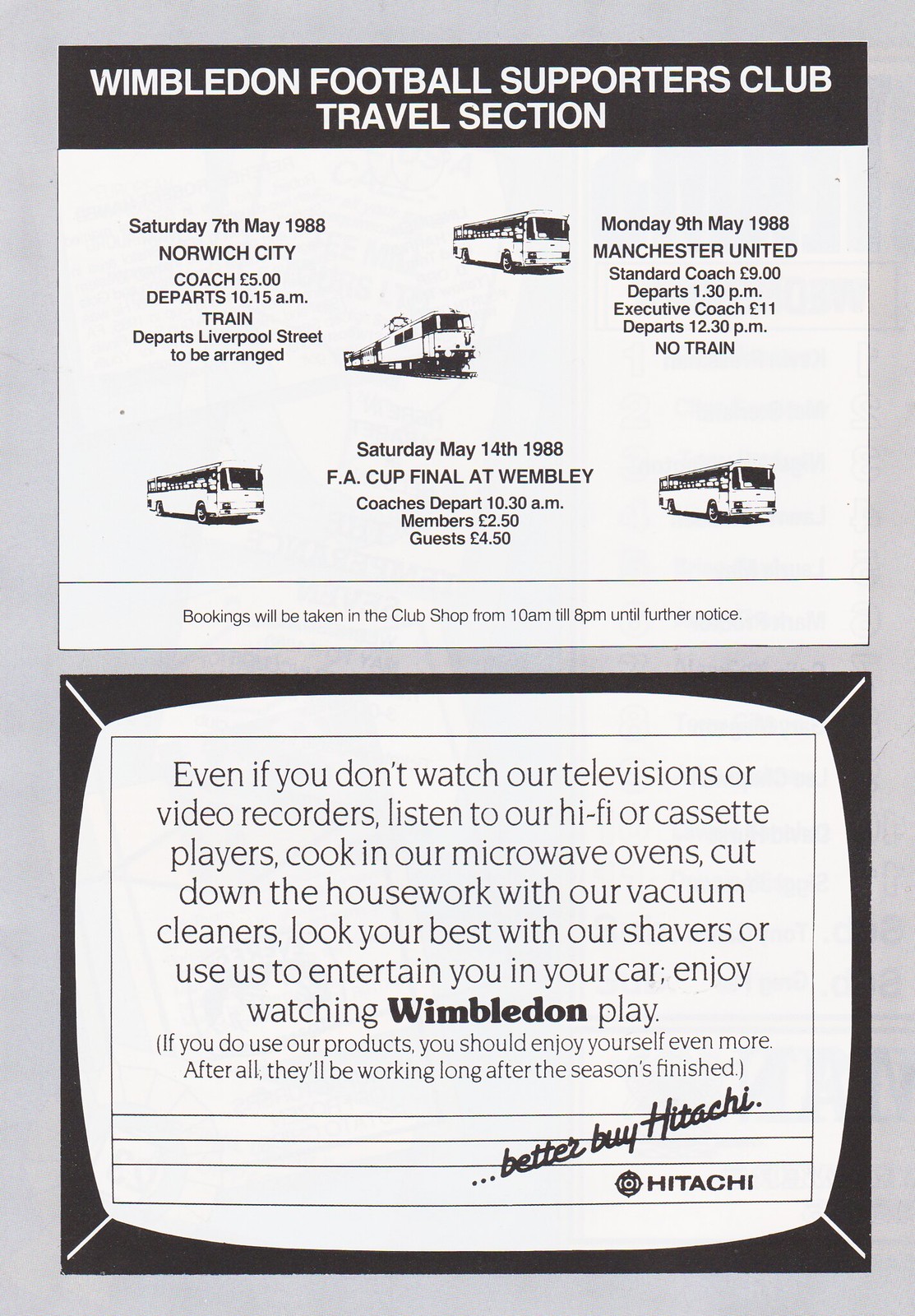This black and white newspaper clipping features a two-part advertisement. The upper half promotes the Wimbledon Football Supporters Club Travel Section, showcasing various modes of transportation including three buses and a tram. It provides detailed departure and arrival information for trips to destinations like Manchester United, with different travel options such as standard and executive coaches. The travel section also mentions that bookings can be made at the club shop from 10 a.m. to 8 p.m. until further notice.

The lower half of the clipping is an advertisement for Hitachi, highlighting its range of electronics. It encourages readers to enjoy watching Wimbledon matches on Hitachi televisions and video recorders, listen to their hi-fi systems and cassette players, cook with their microwave ovens, clean with their vacuum cleaners, groom with their shavers, and entertain themselves in their cars. The ad emphasizes the versatility and quality of Hitachi products, creating a nostalgic glimpse into past advertising styles.